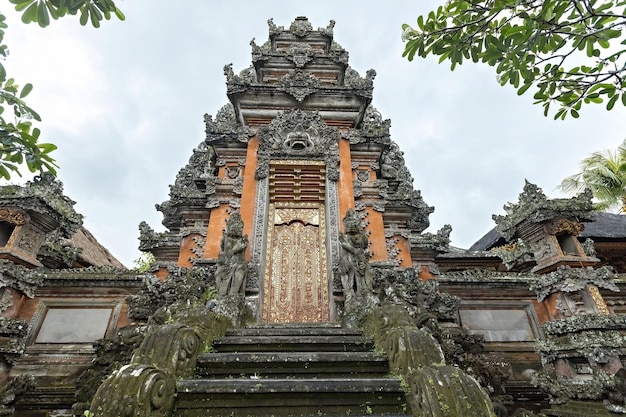This photograph captures the majestic entrance of an ancient Hindu temple in Southeast Asia, likely located in Thailand. The sky above is a clear, brilliant blue, providing a striking backdrop to the temple's intricate architecture. The temple's entrance resembles a small pyramid with steps ascending to a golden, elaborately designed door adorned with vertical Asian script. The pyramid-like structure features ornate carvings, culminating in a rounded triangular apex, rather than a sharp peak. Flanking the entrance are extensions of the temple, including windows that appear to be more modern additions. This blend of historical and possibly contemporary elements creates a visually captivating scene, emblematic of the region's rich cultural heritage.